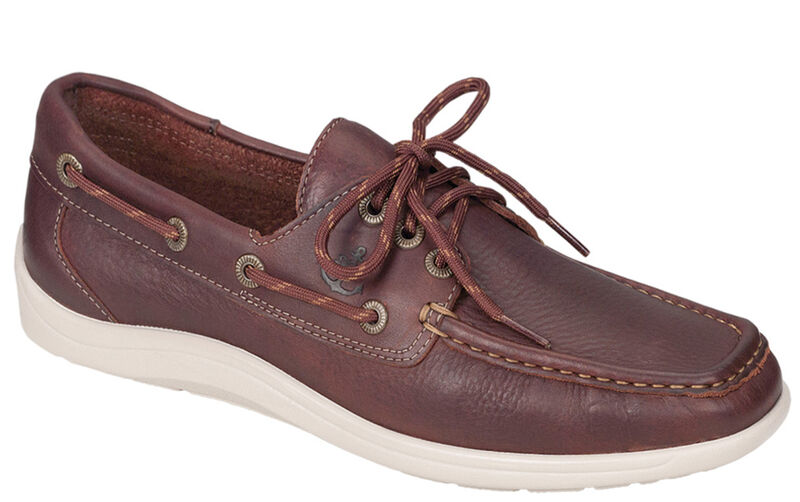This photograph features a meticulously crafted men's leather boat shoe, showcasing an elegant yet functional design. The shoe boasts a rich dark brown leather upper, seamlessly complemented by an off-white rubber sole, which offers both style and comfort. The cream stitching intricately traces the contours of the shoe, highlighting its high-quality construction. Dual lacing details are present: a continuous lace threading around the exterior edge of the shoe and classic laces on the top, resembling robust paracord. Adding a nautical touch, a small anchor emblem adorns the side of the shoe, emphasizing its maritime heritage.